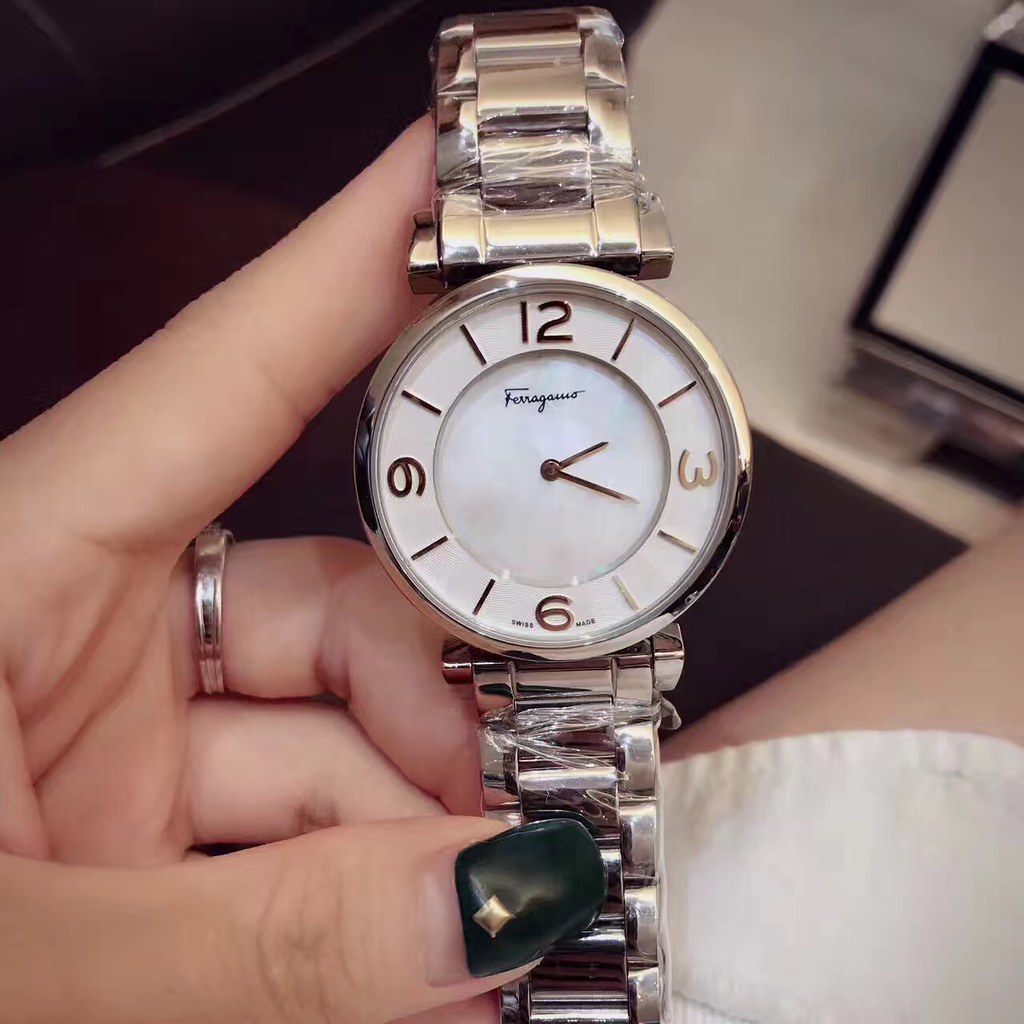In the image, a close-up shot captures a feminine left hand holding a sophisticated silver wristwatch. The hand, emerging from the left side of the frame, has meticulously manicured nails featuring black extensions with a golden diamond at the base. On the middle finger, there's a ring, adding to the elegant aesthetic. The watch itself is an exquisite piece with a metal band and a white clock face that features gold markers for the hours 12, 3, 6, and 9, and simple gold bars for the other hours. The hands of the clock are also gold, indicating the time is 2:20. The brand name "Feragausso" is written in cursive on the watch face. In the background, a glimpse of the person's leg clad in white clothing and a table can be seen, contributing to the image’s intimate and poised ambiance.